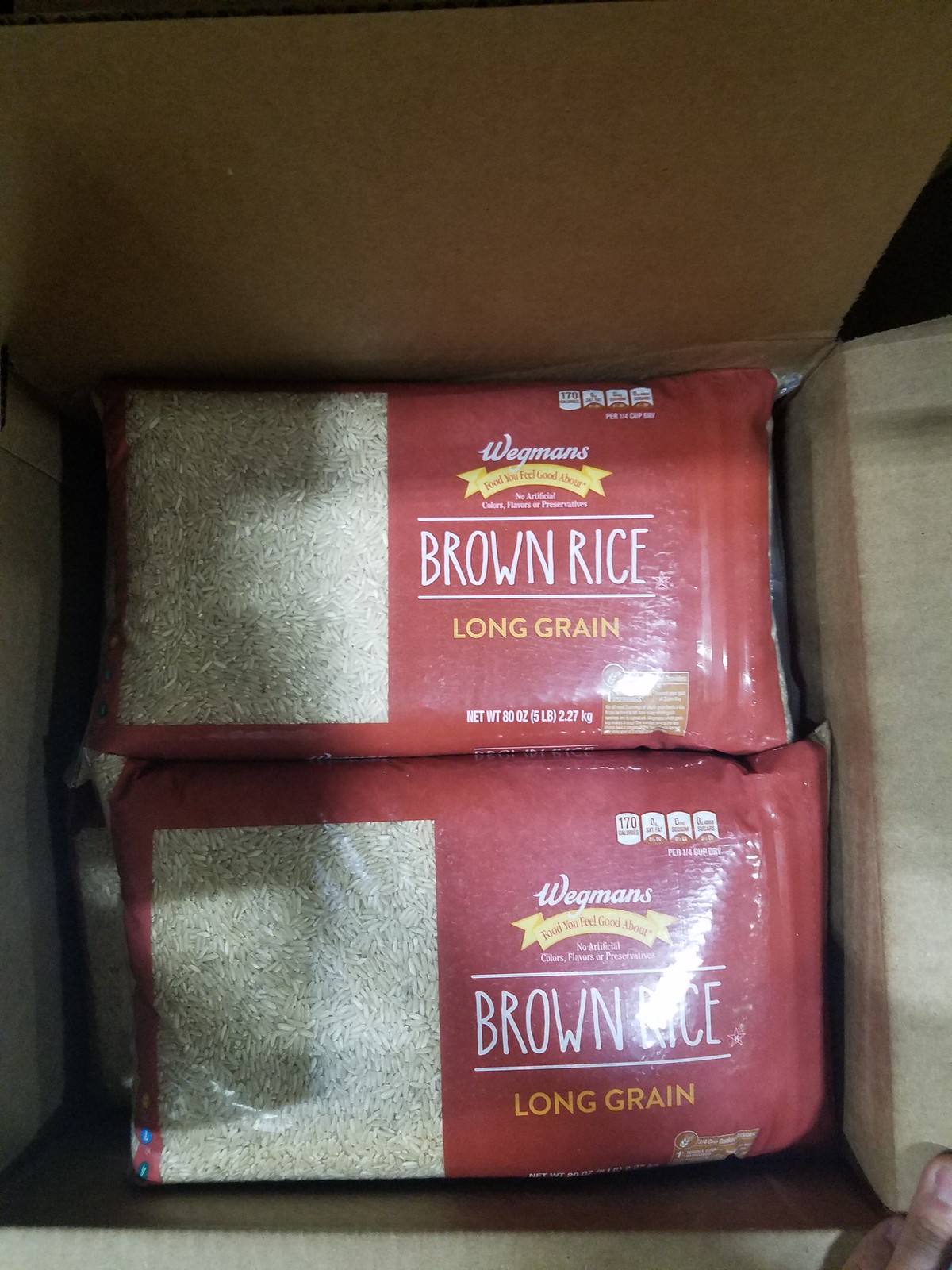The image shows two packages of Wegmans long grain brown rice inside a corrugated cardboard box. The red packages feature a prominent, clear window on the left side that displays the rice grains. At the top of each package, the brand name "Wegmans" is printed, followed by a yellow ribbon that reads "Food You Feel Good About." Below, there is text indicating that the product has "no artificial colors" along with other details. The label includes the text "brown rice" and "long grain" in white and yellow fonts, respectively. The net weight at the bottom of each package states "80 ounces, 5 pounds, 2.27 kilograms." Nutritional information is visible on the top right of the packages. The image captures the packages neatly stacked inside the box, with the carton flaps slightly open, and part of a person's hand is visible in the bottom right corner of the frame.